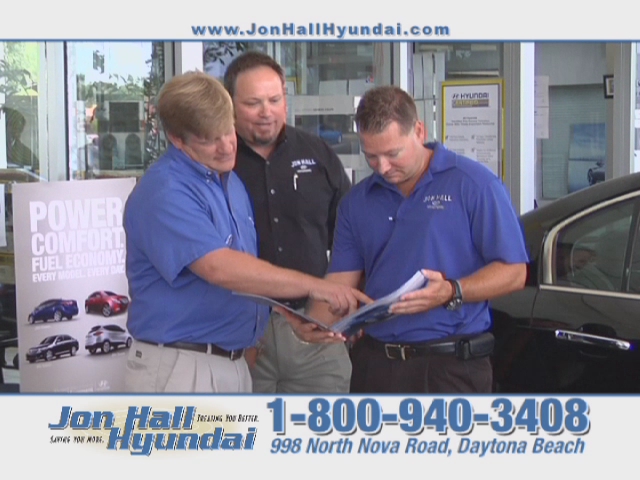In this advertisement for John Hull Hyundai, three men dressed in semi-professional attire—polo shirts and button-down shirts with dress slacks—are engaged in a discussion within a car dealership showroom. One man, wearing a blue polo shirt and black slacks, holds open a catalog or pamphlet, while another man in a light blue button-up shirt and white slacks points to something within it. The third man, standing between them in a black button-up shirt and dark grey pants, observes attentively. All three men have the dealership’s logo embroidered above their shirt pockets. They stand beside a sleek, black car with a visible silver edge on the back door, likely a new model on display. Behind them is a large glass wall that separates the showroom from the sales offices. On the left-hand side of the image, a poster highlights different Hyundai models with keywords like "power," "comfort," and "fuel economy," emphasizing that every model excels in these areas. The text prominently displays the dealership’s website, www.johnhullhyundai.com, and contact information, 1-800-940-3408, along with the address, 998 North Nova Road, Daytona Beach.